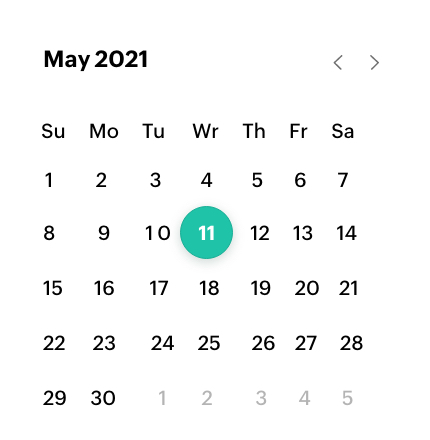The image is a vertically-oriented rectangular calendar set against a solid white background. The header, displayed in bold and larger font, reads "May 2021." In the upper right corner, there are gray left and right arrows, likely intended to navigate to the previous or next month. 

Days of the week are abbreviated in two-letter columns: SU (Sunday), MO (Monday), TU (Tuesday), WE (Wednesday), TH (Thursday), FR (Friday), SA (Saturday). The dates are arranged sequentially from the 1st to the 30th, starting in the upper left corner right below "Sunday." The date numbers are predominantly in black. 

The exception is Wednesday the 11th, which is highlighted with a green circle of slightly lighter than medium shade, featuring the number "11" in white.